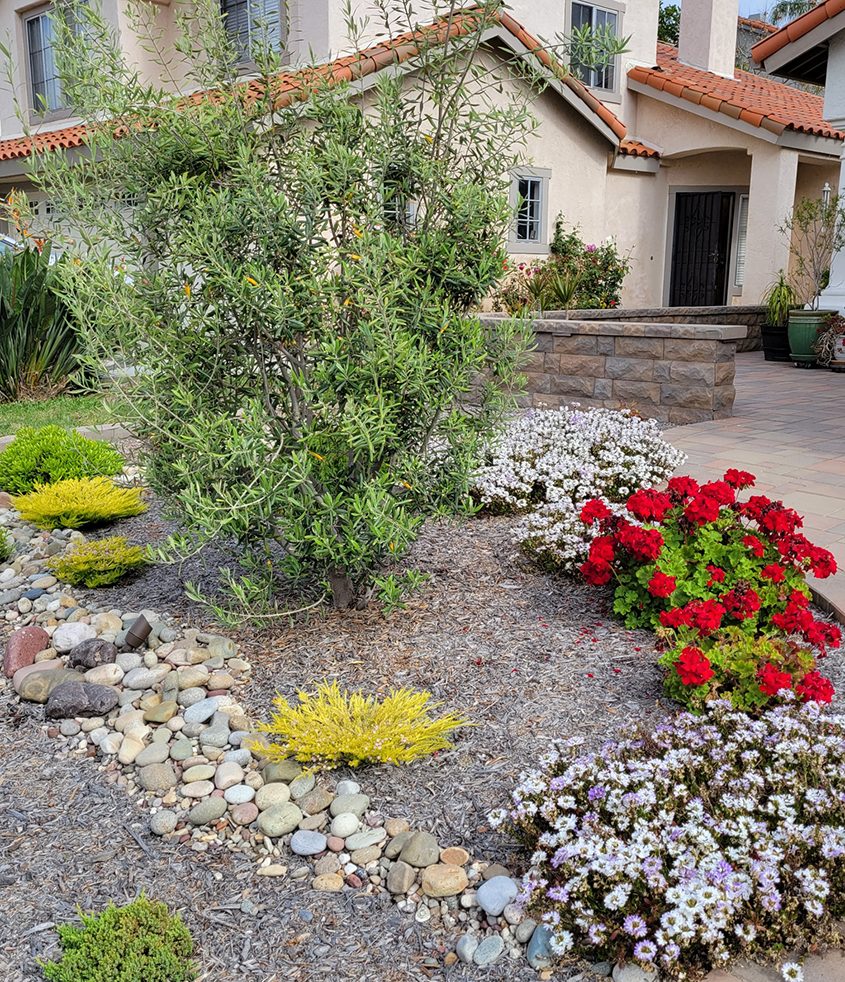This vibrant, close-up color photograph captures a meticulously landscaped section of a chic garden situated in front of a beige-pink stucco duplex house with a red, burnt-orange, and brown tiled roof. The garden is arrayed along a driveway, enveloped by a short slump stone wall. Defined by a curved outline of meticulously arranged white pebbles and a border of lush white flowering plants, the garden features a centerpiece of a large shrub with light green foliage. Scattered around are red, white, and yellow flowers, adding bursts of color against a textured brown mulch surface. In the background, the house stands with its multiple windows on both stories and a brick walkway leading up to a covered entryway, framed by a small cement barrier. The meticulous arrangement and the variety of hues ranging from lilac to shades of purple emphasize the garden's vibrant palette, enhancing the photograph's realistic representation.